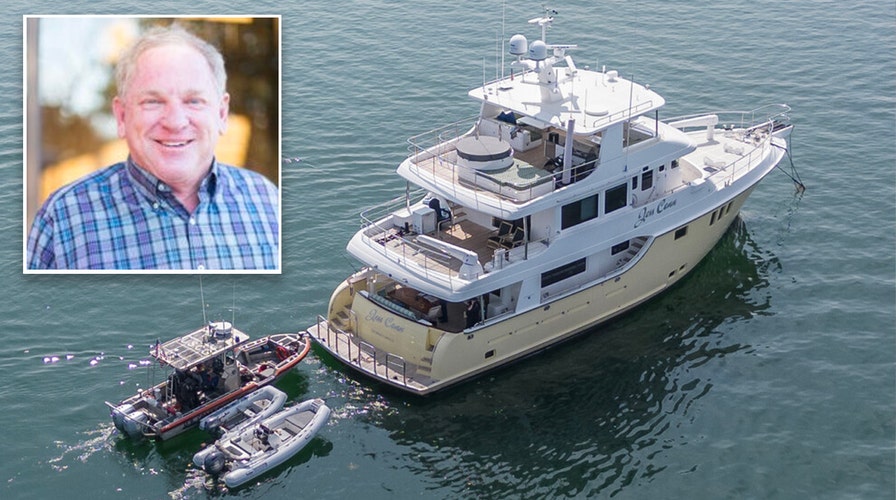In the foreground of this image is a large, classic-looking yacht sailing on a calm, greenish lake under a sunny sky. The yacht, styled in a tannish-yellow and white color scheme, is three stories tall and displays elements reminiscent of designs from the early 1980s. The yacht features a front deck, two back decks with railings, a top roof at the back, a circular gray-topped object, and steps leading to various levels. It also includes multiple rows of windows, antennas, and a distinct yet unreadable name on its rear.

Trailing the yacht are three smaller boats: one primarily white with a red line and simple machinery, and two motorized rafts with one being smaller and the other larger and oval-shaped. The boats are arranged diagonally, with the smaller raft closer to the foreground.

Superimposed in the upper left corner of the image is a photograph of a smiling, gray-haired man, appearing to be in his fifties to seventies. He wears a collared, button-up plaid shirt in shades of white, blue, purple, and black. The man's genuine smile highlights his visible top teeth, and he is illuminated by light coming from the right. Behind him is a grey vertical surface aligned to the viewer's left, faded foliage, sky, and a yellow object in the background. This detailed overlay suggests that the man may be the owner or operator of the yacht, reflecting a personal connection to the scene.